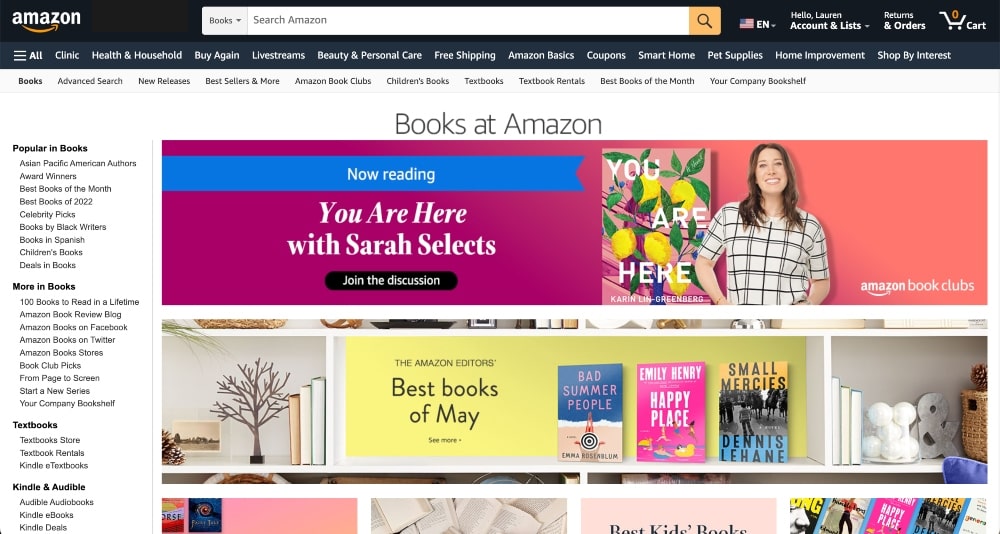The Amazon search result page is displayed, focusing on the "Books" category from a drop-down menu. The search bar at the top reads "Search Amazon." Below it is a highlighted section titled "Book the Amazon," featuring a vibrant purple and pink image. On the left side of this section, a blue ribbon labeled "Now Reading" is prominently displayed, along with the text "You are here with Sarah Selects." Beneath this, a black button encourages visitors to "Join the Discussion." 

To the right, a book is showcased in a pink-themed area. The book title, "You are Here," by Karen Lynn Greenberg, is accompanied by an illustration of a lemon tree branch with five lemons and several leaves. A woman wearing a short-sleeved white shirt adorned with black linear patterns is seen. The section is marked with "Amazon Book Clubs," indicating its affiliation. Below this, the accolade "The Amazon Editor's Best Book of May" is displayed, along with references to other notable books such as "See More," "Bad Summer People," and "Happy Place."